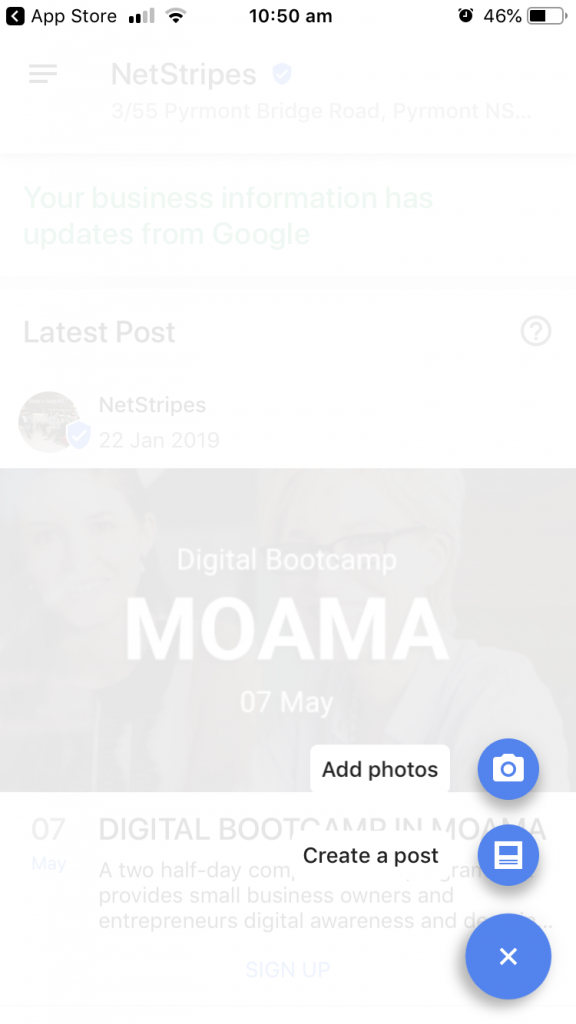This screenshot captures an interface on a website featuring a white background. At the top, there is a black bar containing navigational arrows pointing left and right, labeled "App Store." Adjacent to it, the status bar displays cell signals, Wi-Fi signals, and the time "10:50 AM." Towards the right, it shows an alarm clock icon, a battery icon indicating 46% charge, and the battery's current status.

The website's main content is partially obscured by a pop-up window. The visible portion of the background reveals three horizontal lines with the text "NetStripes" in a capitalized "N" and "S," and the address "3/55 Pyrmont Bridge Road, Pyrmont NSW..." Some of the details get truncated with an ellipsis.

Beneath this, a notification states, "Your business information has updates from Google," followed by the header "Latest post," alongside a circle with a question mark inside it. Below this, it lists "NetStripes" again along with a user profile picture encased in a circle bearing a white check mark on a shield, dated "22 January, 2019."

The main visual content includes a banner or image with the text "Digital Bootcamp Moama" boldly stating the date "07 May" and a follow-up emphasis on "Digital Bootcamp in Moama." 

The pop-up over the background offers two options: "Add photos" and "Create a post." There are corresponding icons for each: a blue circle with a white camera for adding photos, and an icon resembling a laptop screen and keyboard with the same purple-blue color and an X inside it for creating a post.